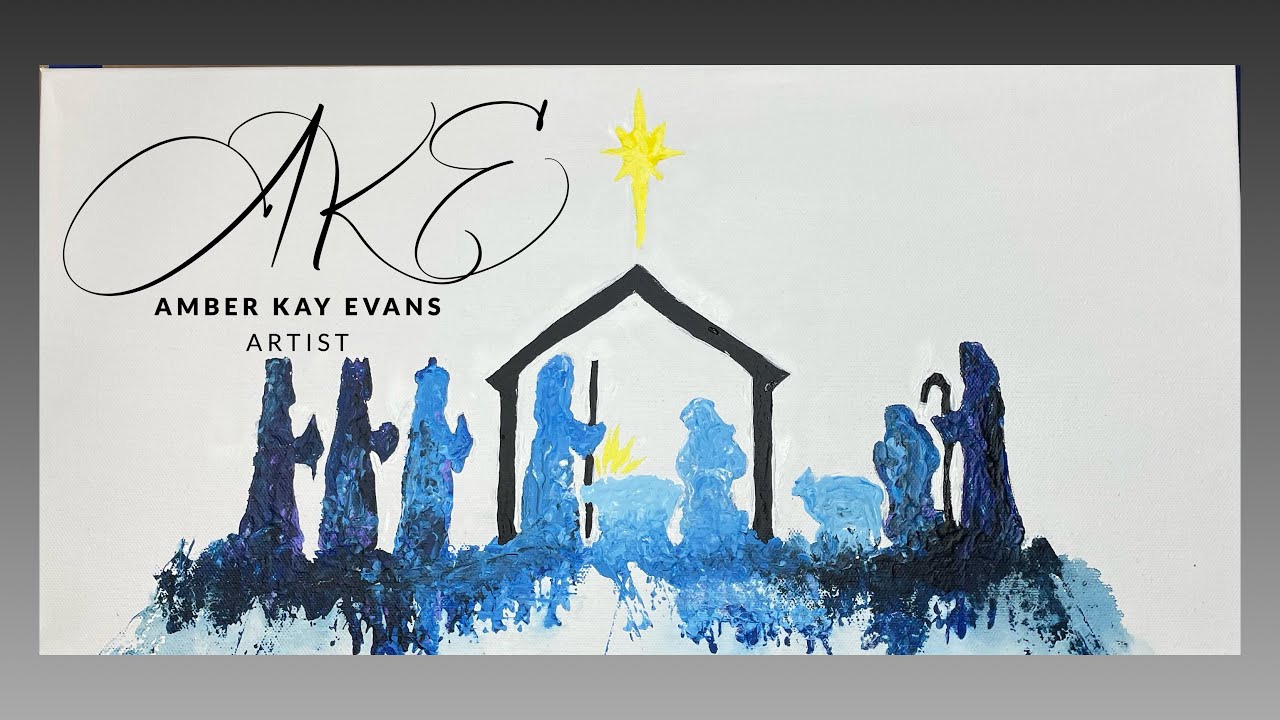This image is a detailed painting of a nativity scene, framed within a rectangular border. The entire artwork measures approximately five inches wide by three inches high, and features a gradient border that transitions from dark gray at the top to light gray at the bottom. Inside this border is another rectangle with a very light gray background. In the upper left-hand corner, in large gray calligraphy, are the letters "A-K-E," and below that, the bold black text reads "Amber K. Evans, artist," identifying the painter.

Central to the art is a stylized acrylic painting of the nativity scene, rendered predominantly in shades of blue, black, and yellow. The scene features a basic, stick-outline manger painted in black or dark gray, resembling a simple house. A brilliant yellow star shines from above the stable, symbolizing the guiding Star of Bethlehem. At the heart of the painting, Mary, Joseph holding a staff, and the baby Jesus in a cradle are depicted in various light blue tones, with a luminous yellow glow emanating from the cradle.

Flanking the central figures, on the left, are the Three Wise Men, painted in shades that transition from light blue to dark grayish purple. On the right-hand side, there is a sheep outlined in light blue, a vague figure in darker blue, and a shepherd holding a curved hook, illustrated in dark grays and purples. The overall composition is blue-shifted, enhancing the serene and mystical atmosphere of this nativity scene.